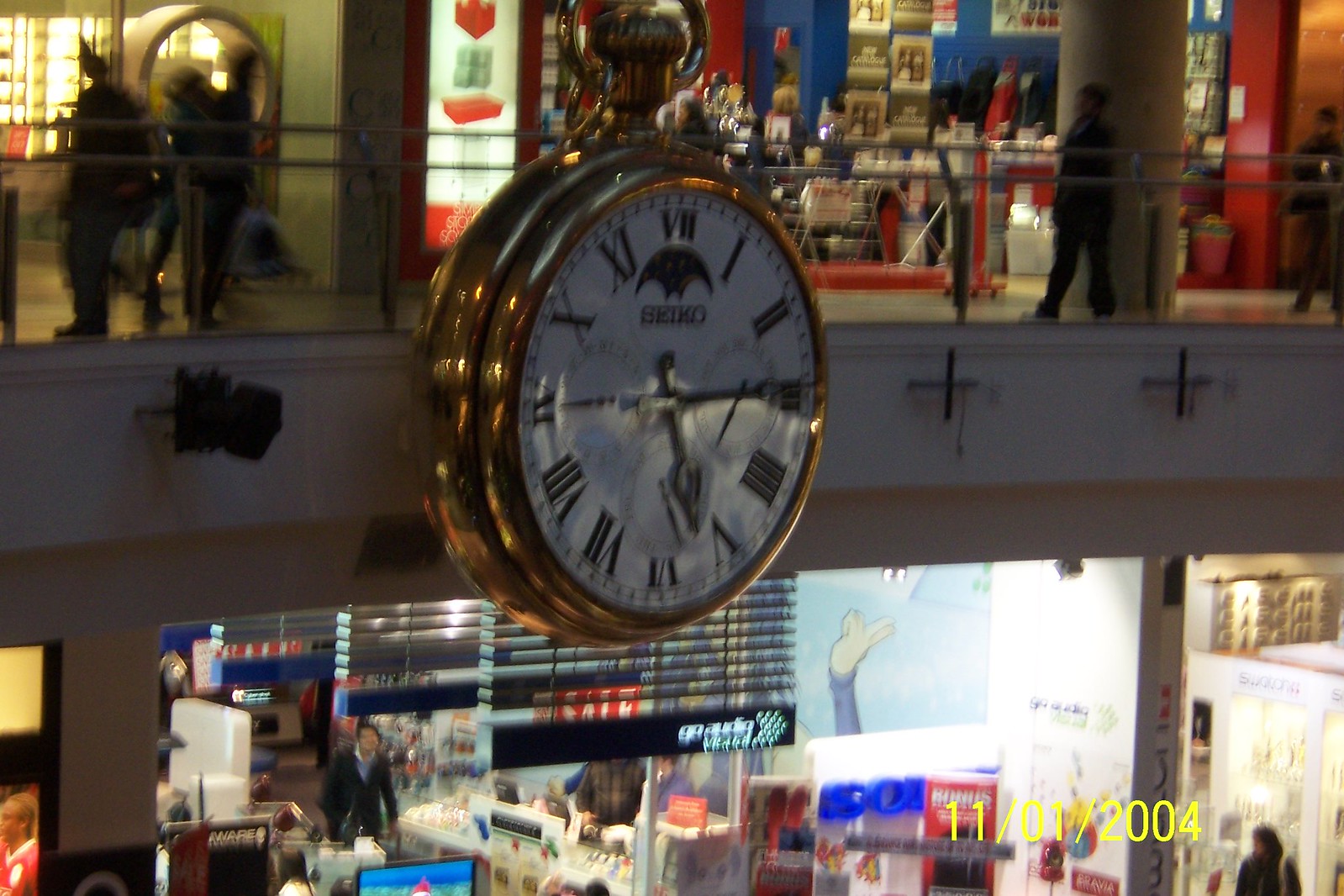The image captures a bustling mall interior from 2004, with an upper and lower level visible. The centerpiece is a massive clock designed to resemble a giant pocket watch, complete with a winding knob, Roman numerals, and a distinctive logo. This clock is attached to a second-floor balcony, appearing gold and intricately detailed. The scene includes numerous shops on both levels, some with Asian language signage, suggesting a diverse retail environment. A security camera is positioned behind the clock to the left. The lower-level stores seem to offer a variety of items from jewelry to technical gadgets, although the image quality is low. The time displayed on the clock is 5:15. The date "11-01-2004" in yellow is visible in the bottom right corner, adding a timestamp to this nostalgic scene.